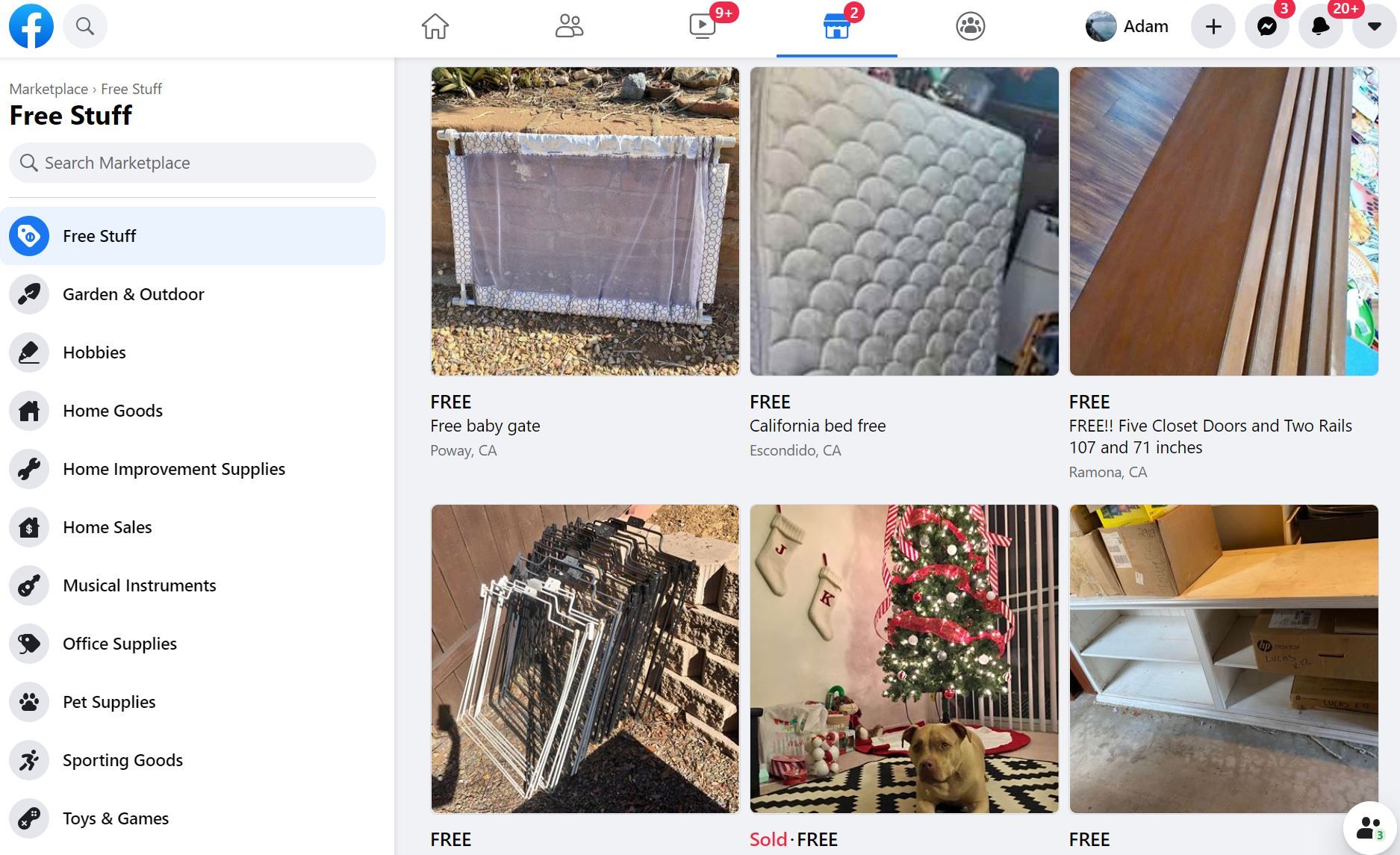In this photograph, Tom Fletcher captures a bustling scene in front of Manifind Glass, a distinctive building known in the community. Friends and passersby gather near Liz's Shop, a quaint and popular local store. The image also subtly highlights Tom's Marketplace, a charming venue offering an eclectic mix of items including musical instruments, office supplies, and pet supplies. The setting is the Texas Garden, an outdoor space where locals engage in a variety of hobbies and home improvement projects. In the background, a cheerful Christmas tree adds to the festive atmosphere. For further details, viewers are encouraged to visit www.facebook.com or www.youtube.com.